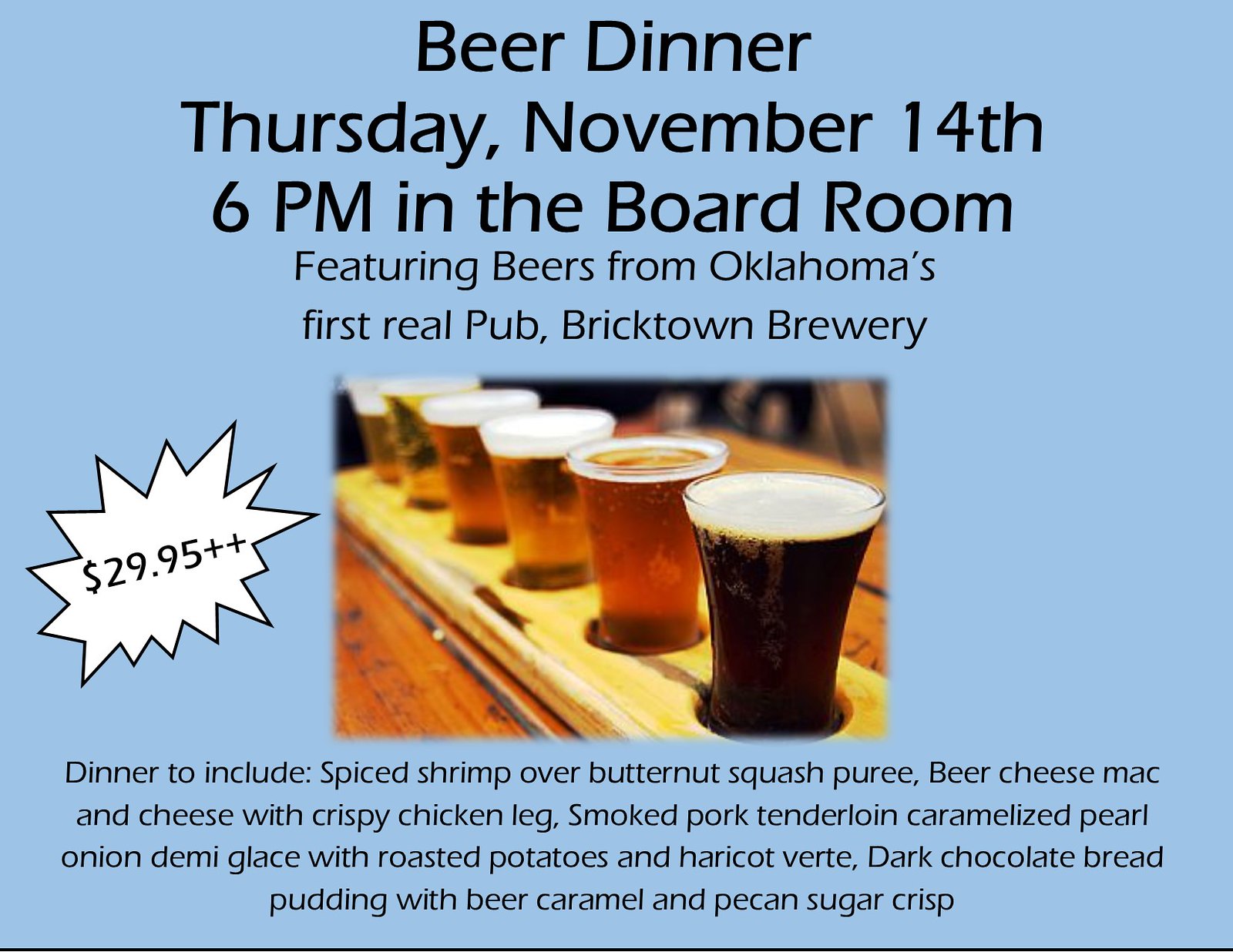The advertisement showcases a special beer dinner event set against a simple, light blue background. Dominating the center is an enticing image of various glasses of beer lined up on a wooden bar. At the top, bold dark text announces the event details: "Beer Dinner, Thursday, November 14th, 6 p.m. in the Boardroom," highlighting that the featured beers are from Oklahoma's first real pub, Bricktown Brewery. On the left side, a white boom logo with a price tag reads "$29.95++." Below, the text elaborates on the gourmet offerings for the evening: "Dinner to include spiced shrimp over butternut squash puree, beer cheese mac and cheese with crispy chicken legs, smoked pork tenderloin with caramelized pearl onion demi-glace, roasted potatoes and haricot vert, and for dessert, dark chocolate bread pudding with beer caramel and pecan sugar crisp."